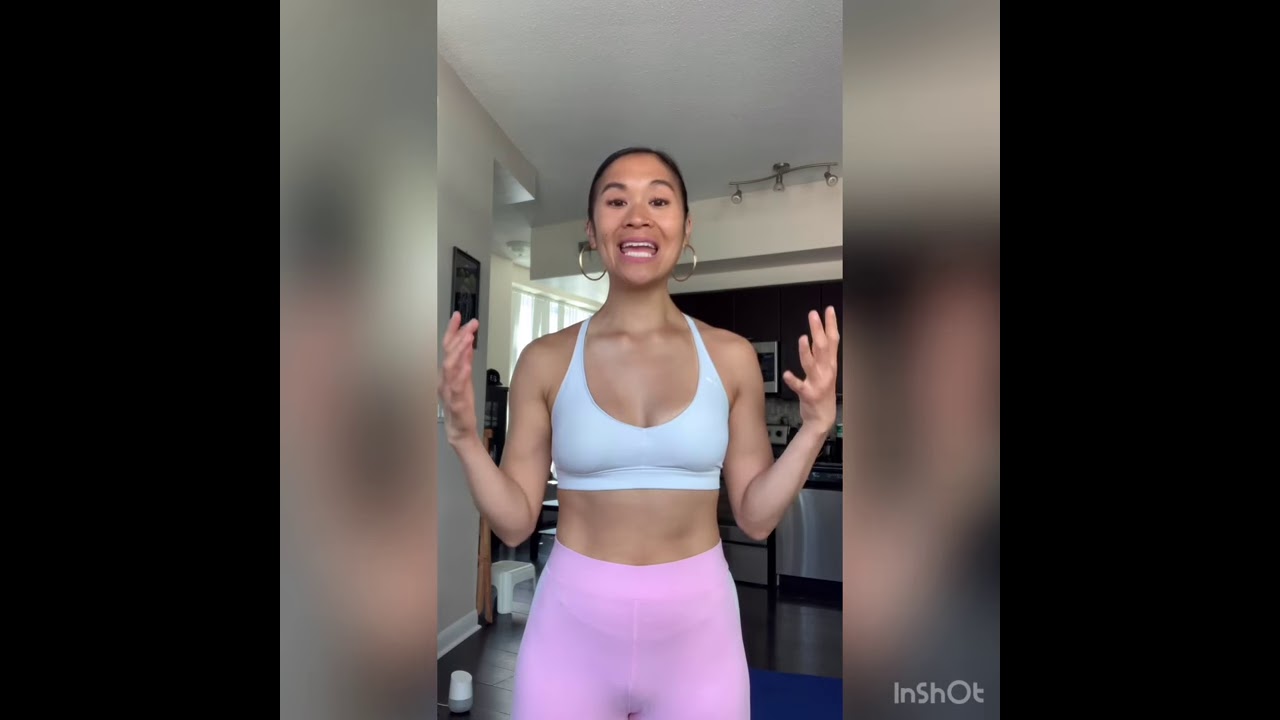In the indoor photograph, an Asian woman with sleek, dark hair pulled back is prominently featured. She sports a padded light gray sports bra paired with high-waisted pink leggings that cover her belly button, showcasing her well-defined ab muscles. The woman stands with both hands elevated above her shoulders, palms facing each other, as if gesturing or demonstrating an exercise. Her expression is lively, with an open mouth revealing white teeth, suggesting she is mid-speech, possibly recording a video or selfie. She accessorizes with large gold hoop earrings. The background reveals white walls adorned with a mounted painting and track lighting suspended from the ceiling, adding a touch of modernity to the setting. To the sides, darker panels frame the central image, and additional details such as a visible stovetop, cabinetry, and a window suggest a multifunctional room. The bottom right corner of the image contains the text "in shot," indicating the photo's alignment within a larger composition.